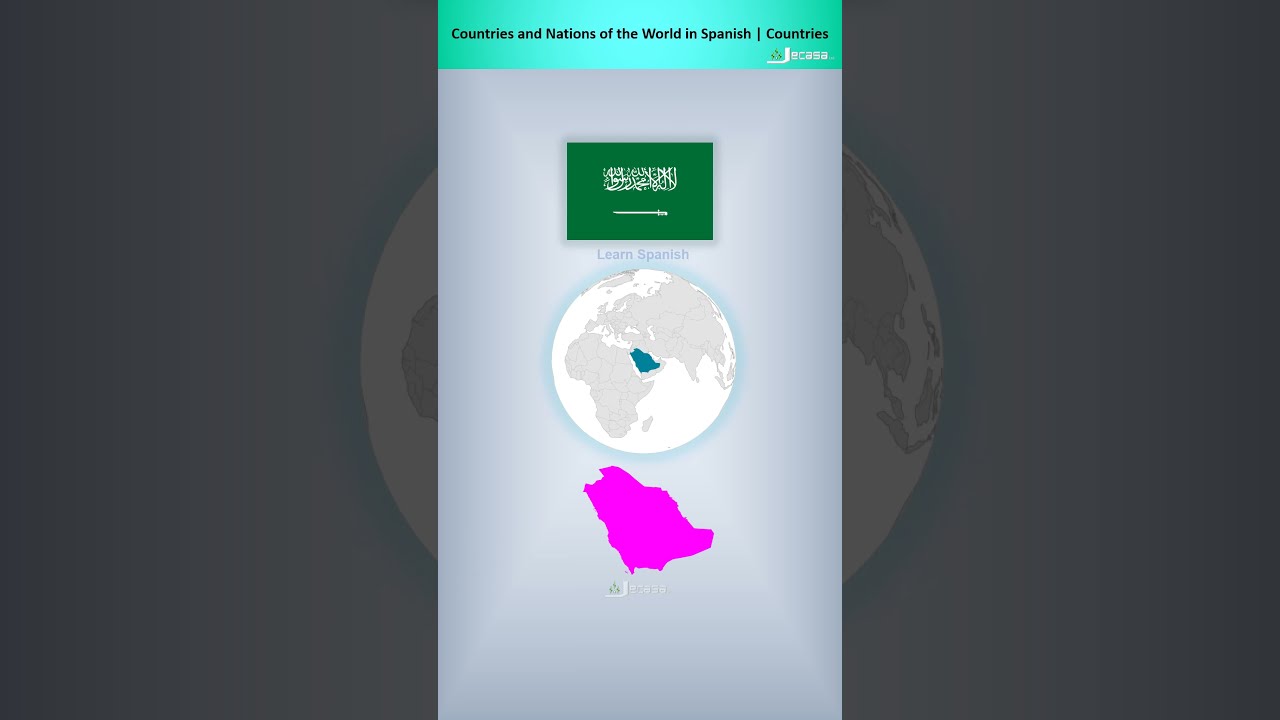The image depicts a digital screenshot, seemingly from a mobile language-learning app. Dominating the central part of the dark gray background is a vertical rectangular box featuring a detailed world map. At the top of this box, a prominent turquoise banner displays the text "Countries and Nations of the World in Spanish." Directly beneath this, a green box instructs viewers to "Learn Spanish." The globe in the center of the screenshot is primarily white with light gray continents. Below this global image, a pink silhouette of a country or continent is highlighted. The color palette includes turquoise, green, light blue, white, gray, black, and hot pink accents. The digitally-created elements provide a sleek, modern look typical of educational app interfaces.